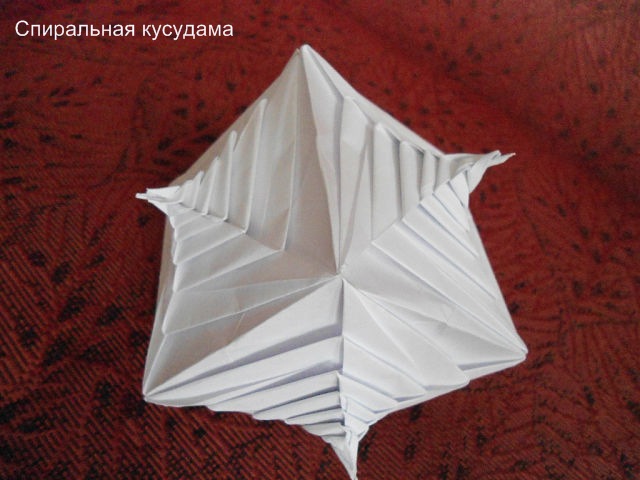This image shows an intricate white star-like figure, carefully crafted with many folds, possibly from paper or fabric. The star, featuring five or six points with a pointed roof-like appearance, is positioned on a textured red and black speckled background, which resembles a cloth, perhaps a sofa. The star stands out in contrast to the vivid background. In the upper left corner, there is some white text in Russian, adding an international element to the design. The photograph, wider than it is tall, captures the complexity and artistry of the star and the detailed texture of the red background.